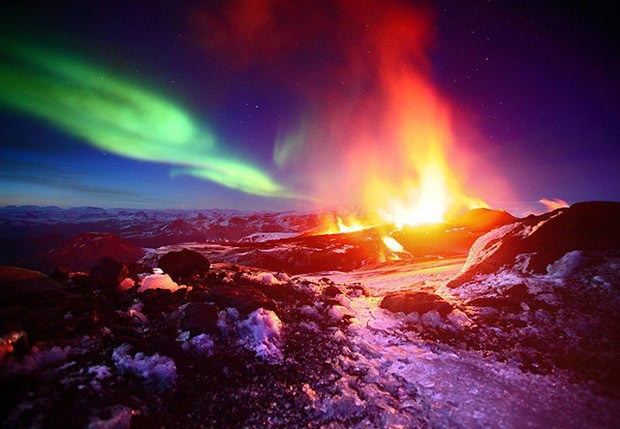The image is a breathtaking, hyper-realistic depiction of a night scene that combines natural elements with surrealistic enhancements, likely created through graphic design or computer AI. Dominated by a dark blue and violet sky, the scene features a stream or rockway at the edge of an ocean or waterway, partially covered in snow or ice, hinting at a winter setting. The main lower half reveals a barren landscape peppered with rocks and craters, resembling another planet. On the horizon, rocky areas meet the remnants of an evening sky, tinged with faint blue.

A striking light show illuminates the scene with fluorescent lime green streaks reminiscent of the Northern Lights, interspersed with small stars. Two dominant, colorful areas descend from the sky: a blue rectangle on the left and an orange-yellow section that merges into the road or landscape below. In the center of the image, a blazing fire creates a vivid focal point. Its bright yellow, nearly white flames transition to red and orange as they ascend, casting a warm glow on the surrounding terrain and intensifying the violet hue of the night sky above. The overall composition is a captivating blend of natural beauty and imaginative artistry.